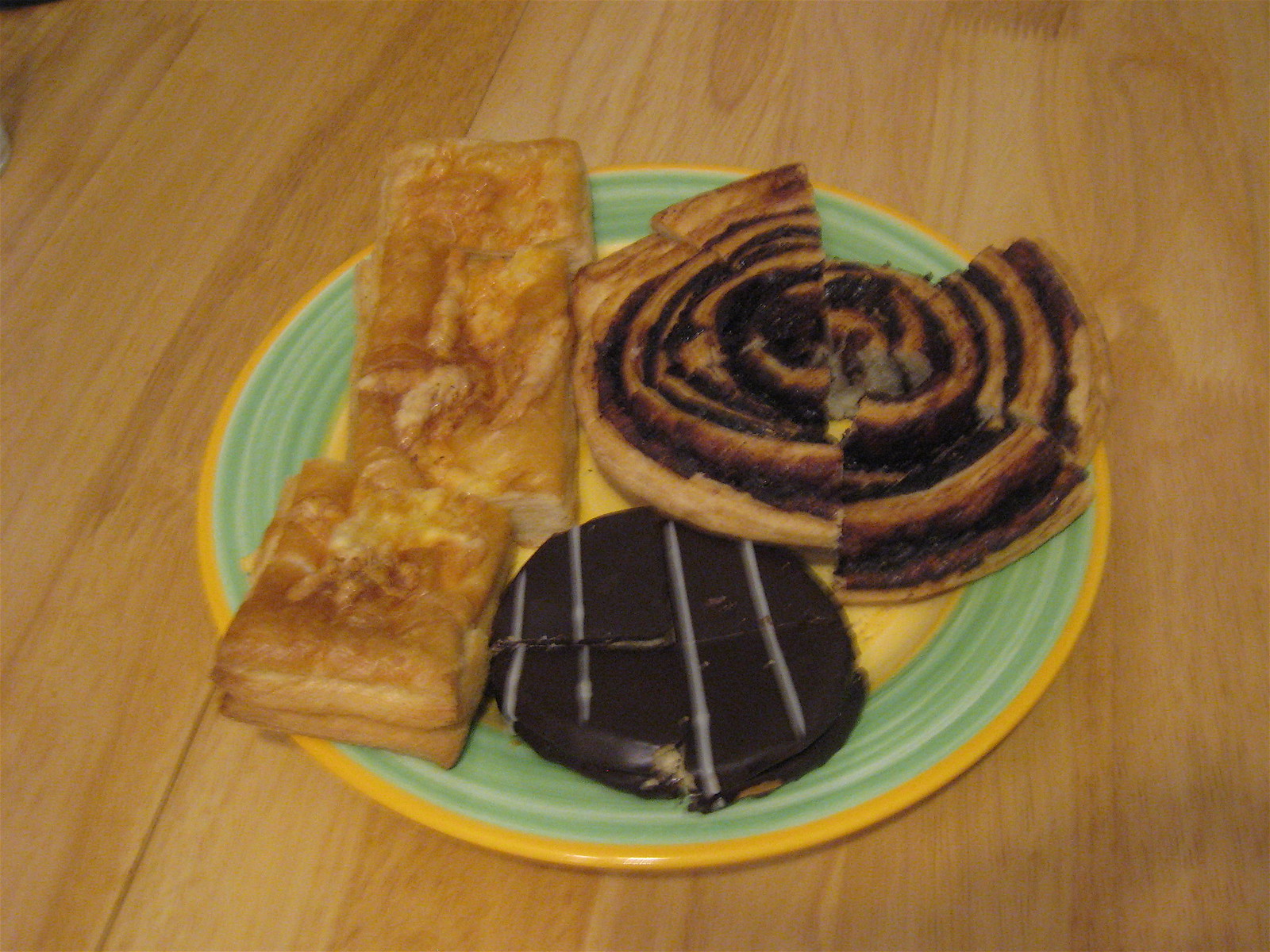A blurry photograph captures three different desserts on a vibrant ceramic plate, which is placed on a light brown wooden surface. The plate itself features a distinctive design, with a bright yellow center, a wide band of light green swirly stripes, and a golden yellow edge. On the left side of the plate rests a rectangular, golden-flaky pastry that appears to be cut into smaller pieces. To its right, at the upper part of the plate, there's a cinnamon roll sliced into multiple pieces, marked by its swirled appearance with a mix of dark brown and beige hues. Below the cinnamon roll, a smaller round chocolate dessert with four horizontal white chocolate stripes is visible; it seems to be cut in quarters. The combination of these various treats on the decorative plate creates an inviting, albeit slightly unclear, tableau of baked goods.